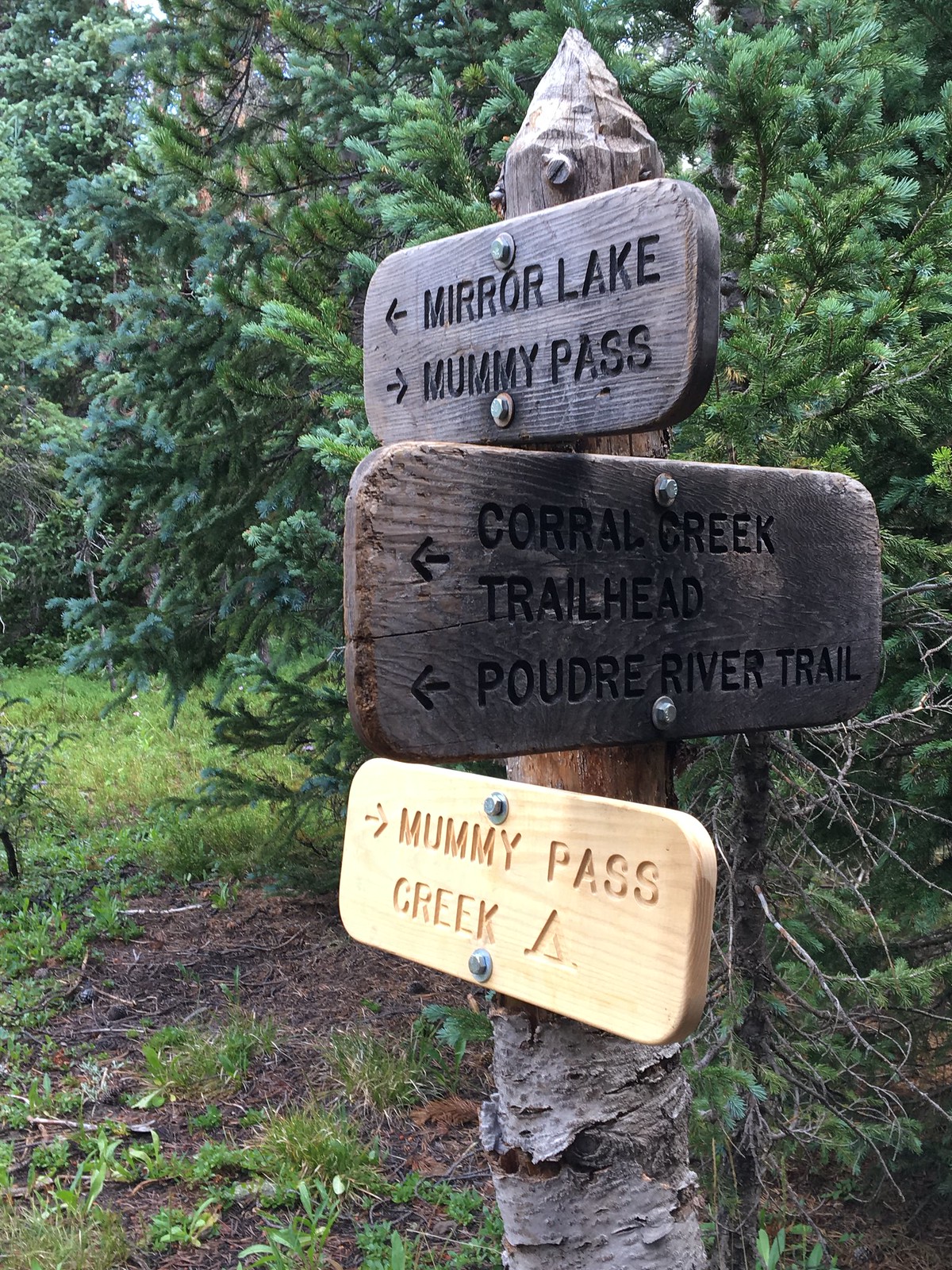The image captures a rustic trail marker in the middle of a dense, daytime woodland. The focal point is a carved tree stump shaped into a pointed post, adorned with three distinct wooden signs. Surrounding the stump are various trees, one of which resembles a Christmas tree, along with lush grass extending into the background.

The top sign, bearing a dark brown hue, features arrows indicating directions: "Mirror Lake" to the left and "Mummy Pass" to the right. Below it, another dark brown sign directs hikers to "Coral Creek Trailhead" and "Poudre River Trail," both with arrows pointing to the left. The bottom, cream-colored sign repeats "Mummy Pass" to the right and adds "Creek" with a small triangle symbol underneath.

This scene encapsulates a serene yet informative trailhead in the heart of nature, guiding adventurers to various destinations within the forest.